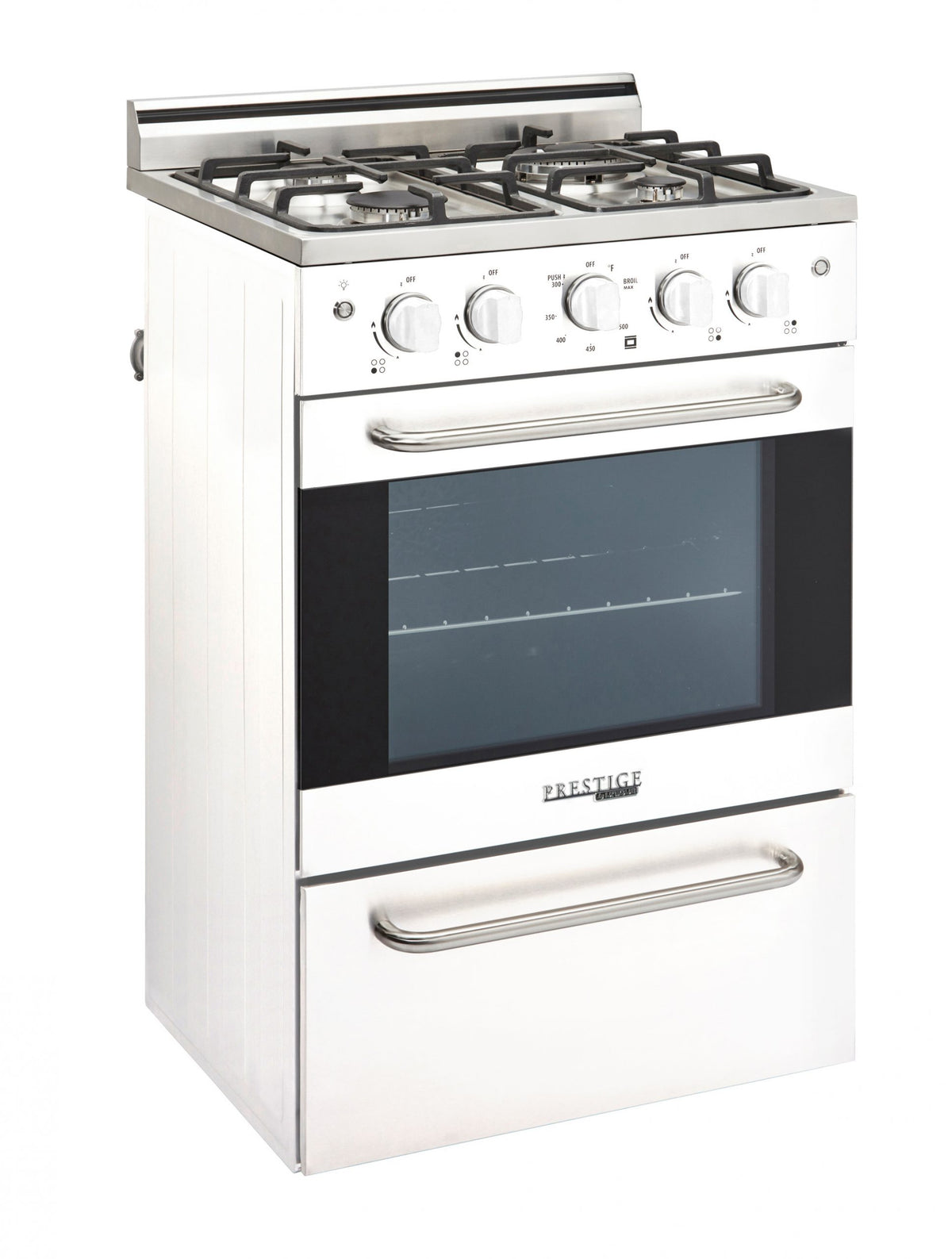This product photograph showcases a Prestige stainless steel gas range and oven set, designed for online commercial listings. The image, with a clean, solid white background, gives the effect of the appliance floating in an empty white void, emphasizing its sleek, modern appearance. The rectangular photograph, twice as wide as it is tall, centers on the silver oven made of polished stainless steel. 

At the top of the appliance are four gas burners, equipped with black support arms for pots and pans. In front of these burners, there are five white control knobs for adjusting the flame, along with two buttons on either side of the knobs. The left button features a small light bulb symbol, presumably for the oven light. The front of the oven has a large, clear glass window allowing a view into the oven's interior, which contains at least one baking rack. The oven door has a prominent stainless steel handle for easy opening. Below the window, the brand name "Prestige" is visible. Beneath the oven door is a large drawer, likely a broiler, which also features a long, silver handle.

The sides of the appliance have vertical striped detailing, adding a touch of style to its functional design. This high-quality commercial product photo highlights the range and oven's features and aesthetic, making it ideal for shops, catalogs, or websites.